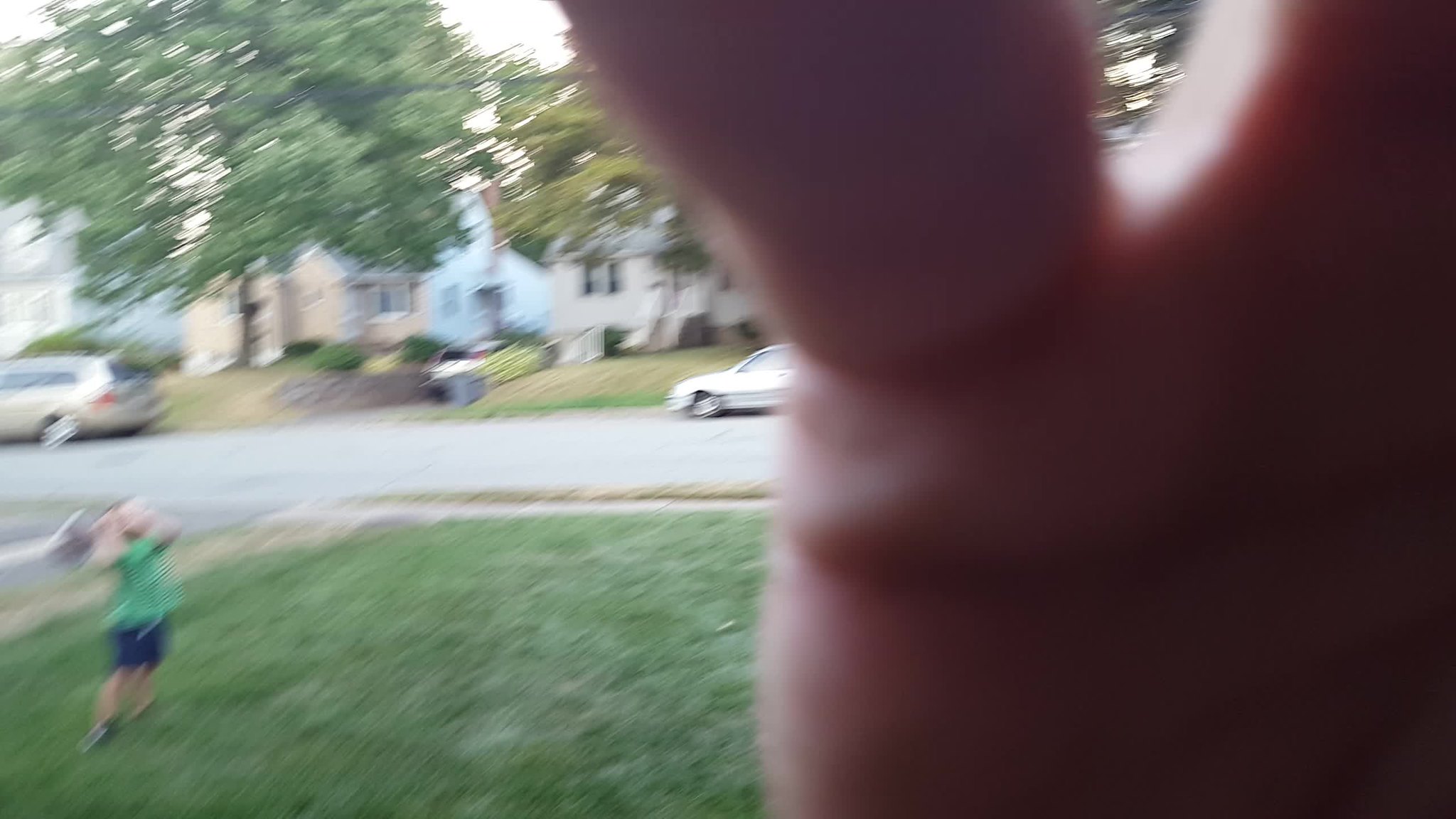This color photograph, taken outdoors during the day, captures a serene suburban scene from the perspective of someone on a porch or near the front of their house. On the left side of the image, a young child wearing a green shirt and blue shorts plays on the grass. The background reveals a residential street with houses and a couple of parked cars. Several mature trees with lush foliage stand proudly across the street, adding to the neighborhood’s picturesque charm. Unfortunately, the right side of the photo is obscured by the photographer's hand, making the image appear blurry and lacking sharp details in that area.